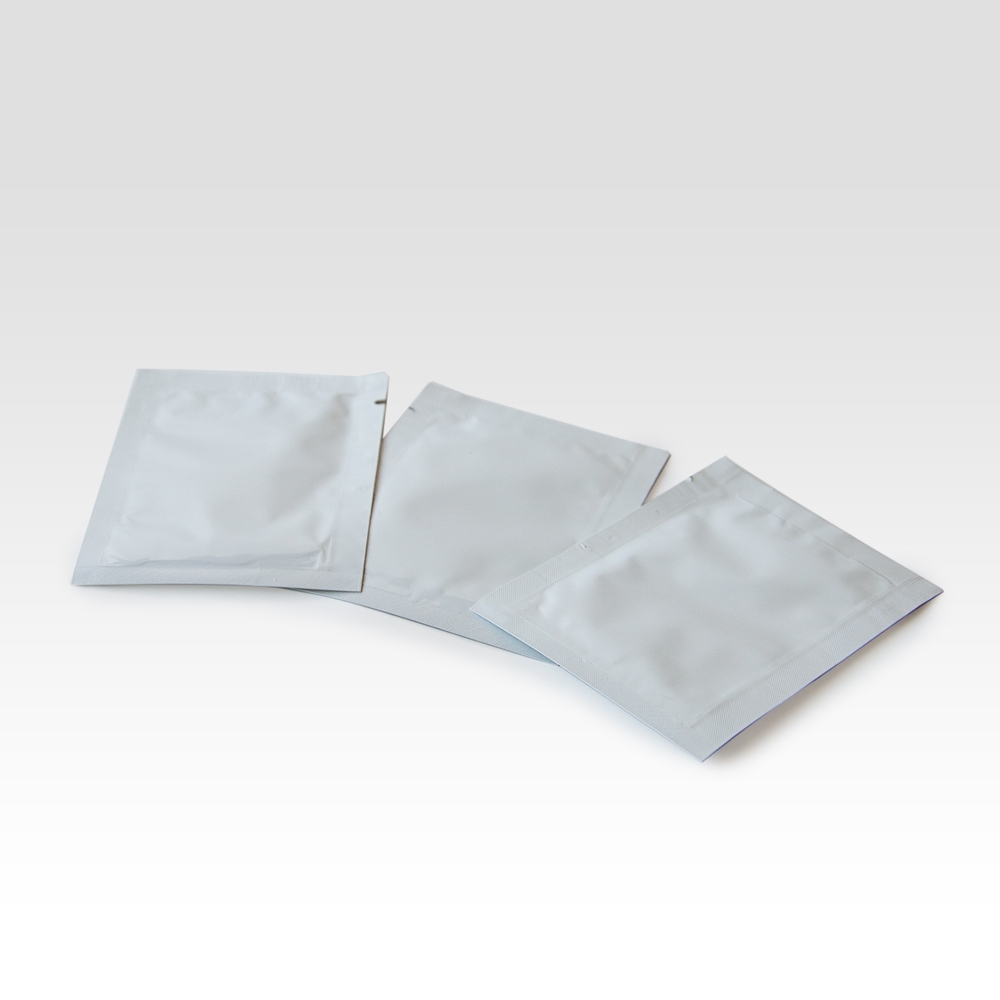This image displays three slightly wrinkled, flat gray plastic packets laid diagonally on a light-colored background, possibly white or light gray. The packets have small tab notches at the top right for easy tearing. Positioned in the center of the image, the leftmost packet overlaps the middle one, while the right packet partially overlaps the middle one but not the left. These packets resemble small, smell-proof bags commonly used at dispensaries or for other supplements and could also be likened to wrappers for individual wet wipes or similar small disposable items. There is no text or markings on the packets, and the overall scene suggests a stock photo or clip art style with only shades of gray and off-white present.